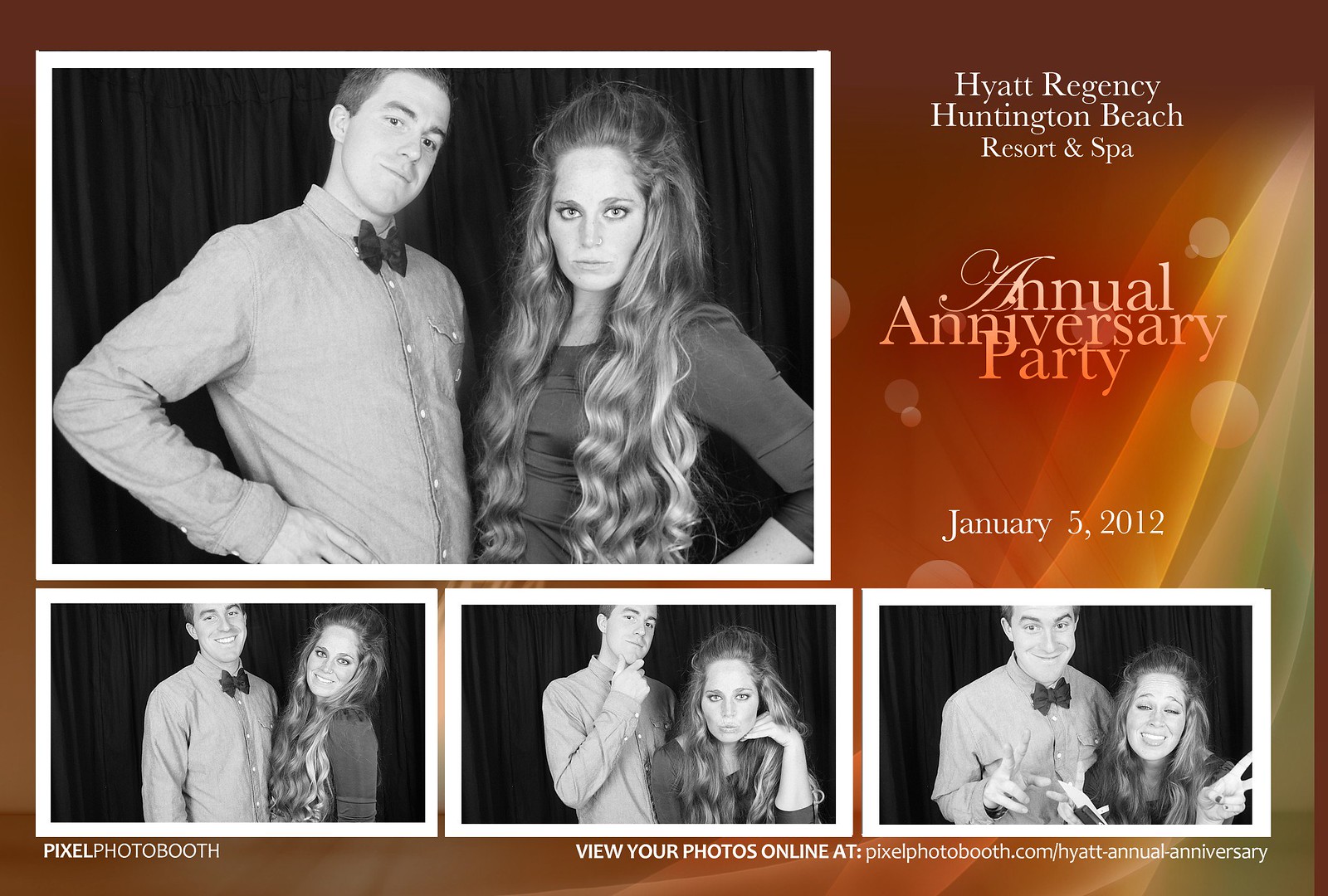The image is a rectangular invitation for the Hyatt Regency Huntington Beach Resort and Spa's annual anniversary party held on January 5, 2012. The background features a warm brown and gold gradient with stylish circles and waves, with beams of light in the upper right corner. The text, styled in both script and serif fonts, reads: "Hyatt Regency Huntington Beach Resort and Spa Annual Anniversary Party January 5, 2012."

At the upper left, there's a large black-and-white photograph of a man and a woman posing seriously and looking directly at the camera. The man has short dark hair, is wearing a bow tie with a button-down shirt, and has his hand on his hip. The woman, with long, wavy hair and bangs styled into a high wave, also has her hand on her hip. Below this main image are three additional black-and-white photos of the couple with white borders, all against a dark curtain backdrop. 

1. The first photo on the left shows them smiling with their heads tilted back and their chests close together, although the man's head is slightly cut off.
2. The middle photo features both with hands on their chins; the man appears contemplative while the woman makes a pouty or kissy face.
3. The final photo on the right captures them making silly faces with peace signs; the man has his eyes open while the woman’s are closed.

At the bottom, there's text that reads "Pixel Photo Booth" on the left and "View your photos online at pixelphotobooth.com/hyatt-annual-anniversary" on the right.